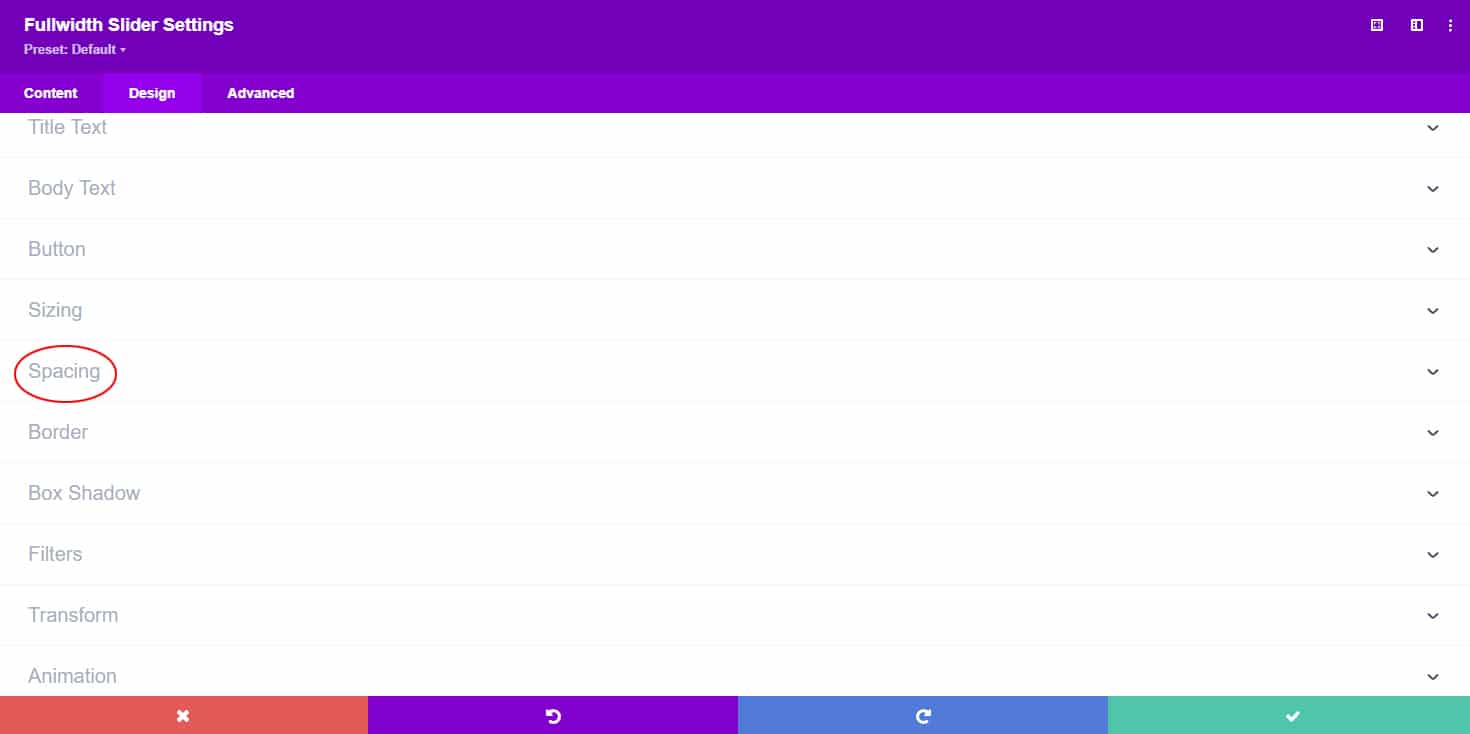Detailed Caption:

The image displays a web page or computer setting interface titled "Full Width Slider Settings," prominently highlighted in white text within a purple bar at the top of the page. Below this bar, the phrase "Preset Default" is visible, indicating the current configuration setting. The interface is divided into three sections: Content, Design, and Advanced, with the Design tab currently active. Within the Design tab, a large white space presents various customization options in gray font, listed as: Title Text, Body Text, Button, Sizing, Spacing, Border, Box Shadow, Filter, Filters, Transform, and Animation. Notably, the "Spacing" option is encircled by a red oval, drawing attention to it. Each option has a corresponding drop-down menu, with clickable arrows located on the far right side of the page.

At the bottom of the page, a thin bar features four evenly spaced, colored boxes, each serving a specific function. The red box, marked with an X, likely serves as a cancel or delete button. The purple box, featuring a swirly back arrow, suggests an undo function. The blue box, showing a swirly forward arrow, represents a redo function. Finally, the green box, adorned with a checkmark, denotes a save or confirm button.